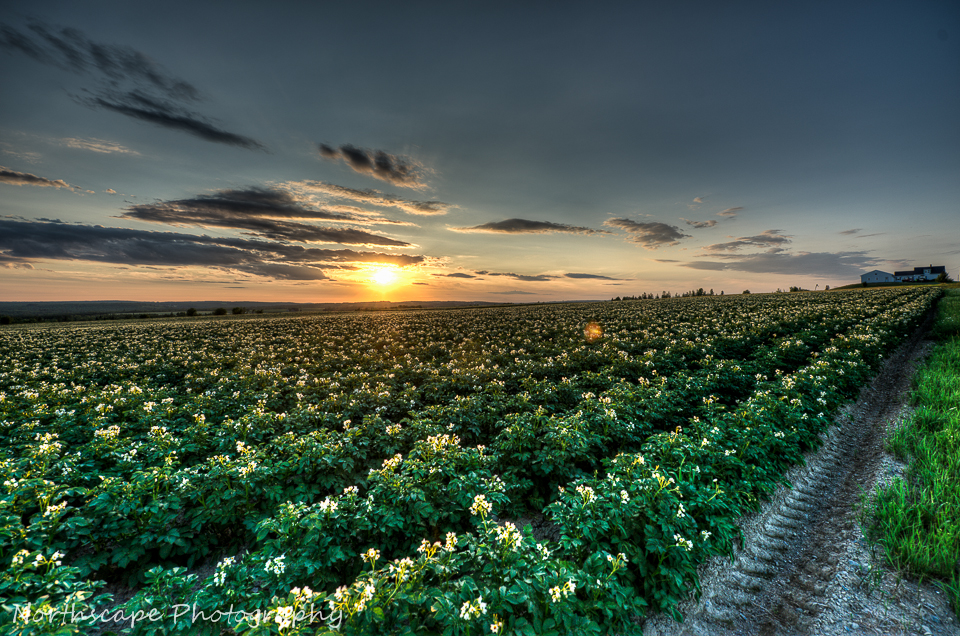In this striking photograph, the viewer is greeted by a sprawling farmer's field, meticulously plowed into neat rows and adorned with green plants boasting white and yellow flowers. A tractor's path, marked by deep wheel imprints, runs from the front to the middle of the field, adding a rustic charm to the scene. Set against a dramatic gray sky, pierced with shades of pink and orange from the sun, the image captures the ethereal moment of sunrise, though one might mistake it for a tranquil sunset. To the right, a solitary farmhouse stands, adding a touch of human presence to the vast, nature-dominated landscape. Wisps of gray clouds add depth to the horizon, while a subtle hint of sunlight pierces through, casting a serene glow over the entire scene. The bottom left corner of the image features the elegant white cursive text, "Northscape Photography," completing the composition and crediting the artistry behind the lens.